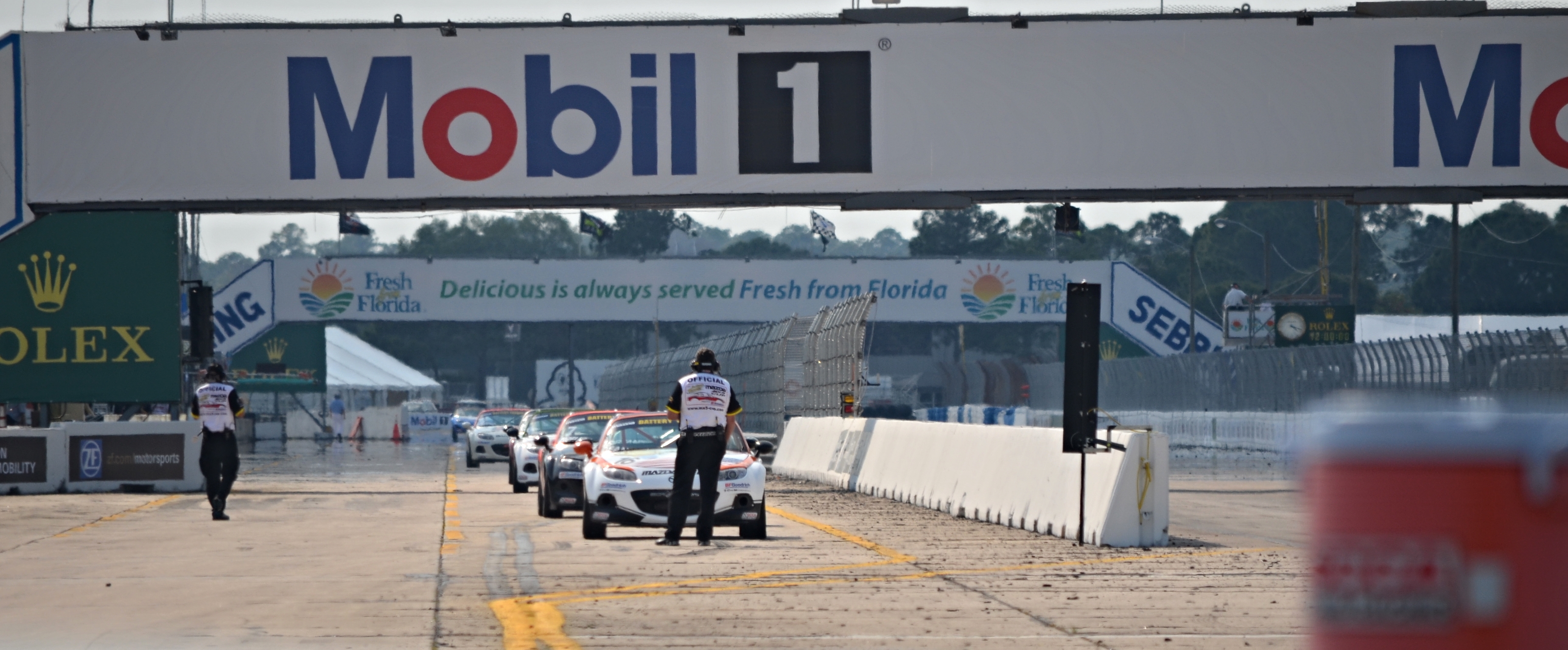The photograph captures a daytime scene at a concrete racetrack, featuring a wide, gray paved area with several professional-looking cars lined up in a single row starting from the center left of the image. In front of the first car, a man dressed in dark pants, a white vest with colorful writing, and a cap, holds light indicators and appears to be giving instructions. Another similarly dressed man stands about 15-20 feet to the left. Both men wear hats and headphones. Overhead, white signage with the word "Mobile 1" spans a large overpass, while nearby banners advertise fresh fruit from Florida and Rolex, among others. In the background, a clear sky and numerous trees frame the scene. Additional elements include green traffic indicators painted on the track, neat central dividers, and a blurred red box in the bottom right corner, as well as a distant clock.